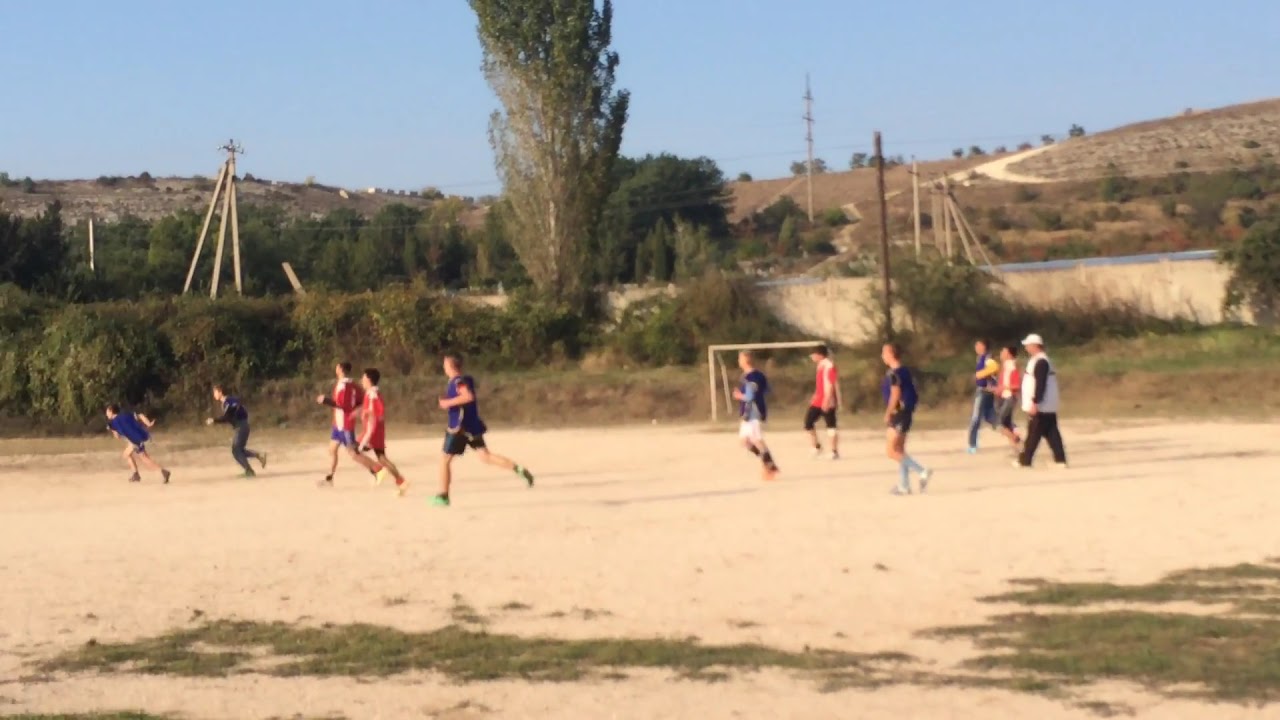In this outdoor image of a soccer game, 11 players are seen on a dirt lot that doubles as a makeshift field. The teams are distinguishable by their colors; one team is clad in blue while the other sports red jerseys. Visible in the scene is a goal post, and a referee dressed in a white overcoat with black sleeves and pants. The image captures players in dynamic motion, heading towards the left side of the goal, presumably chasing an off-frame ball. The terrain features sparse greenery towards the bottom, with some shadows from surrounding trees. In the background, a sloping hill dotted with brown and green vegetation rises, intersected by brown electrical posts holding power lines. A road is faintly discernible, elevated above the field. The sky above is clear and blue with bright sunlight illuminating the scene, setting a vivid backdrop to the energetic game below.